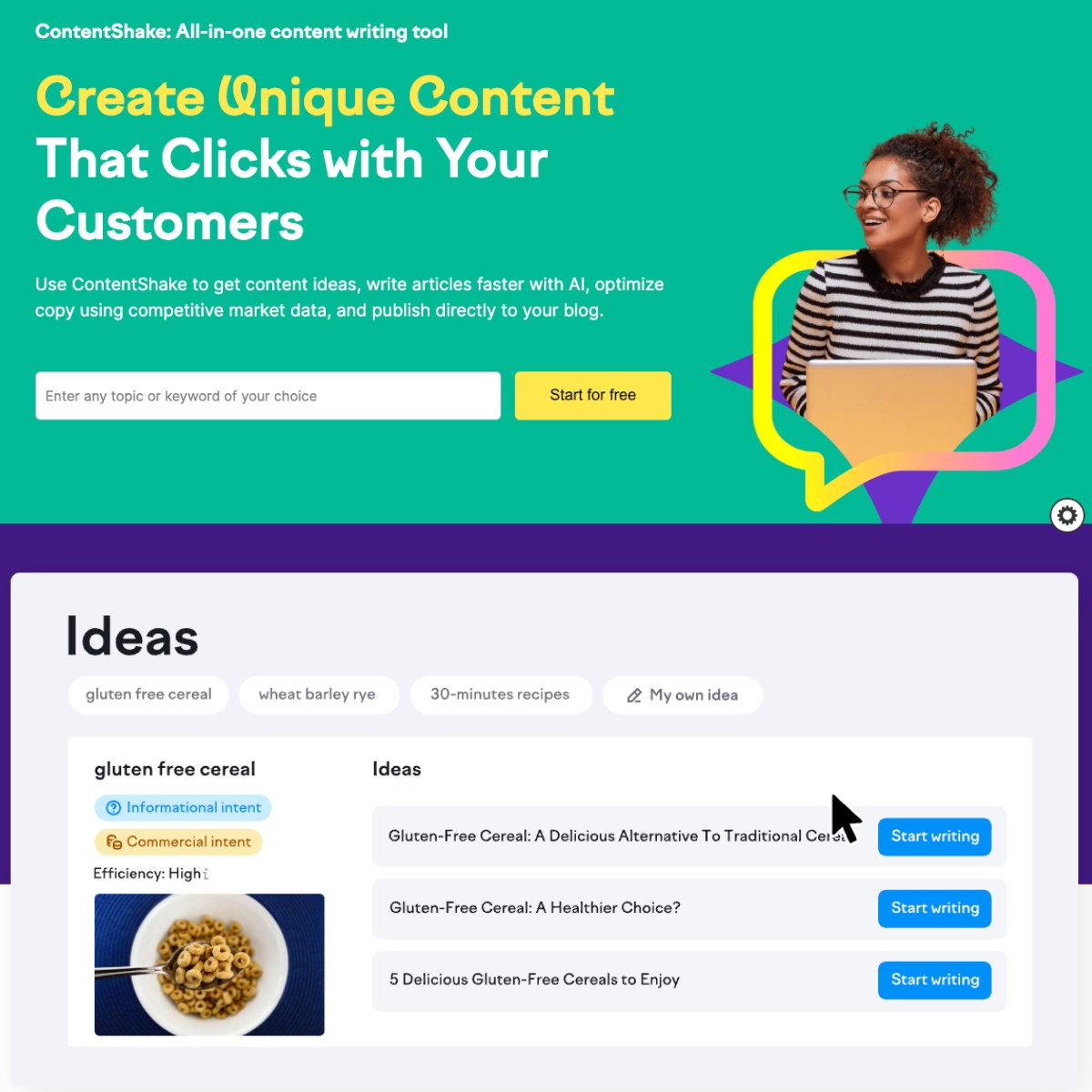**Detailed Caption:**

The screenshot depicts a user interface from an AI-powered content writing application, designed to streamline the process of creating written content. 

*Top Section:* The upper segment features a green background overlayed with prominently displayed yellow and white text. At the very top is the application's logo and name, "Content Shake - All-in-One Content Writing Tool." The subtitle reads, "Create unique content that clicks with your customers." Beneath this tagline, smaller text elaborates on the app's capabilities: "Use Content Shake to get content ideas, write articles faster with AI, optimize copy using competitive market data, and publish directly to your blog." Alongside this informative text, there's a "Start for Free" button, inviting users to begin their content creation journey. Next to the button is a search box labeled "Enter any topic or keyword of your choice," suggesting users can initiate content generation by inputting specific keywords.

*Illustrative Element:* Below the textual information, an image of a woman sitting at a laptop is shown. She appears to be happily engaged in writing, depicted through a speech bubble indicating content production. This visual serves as an idealized representation of the user experience, reinforcing the application's purpose in facilitating efficient and joyful content creation.

*Bottom Section:* The lower half of the screenshot transitions to a white background with a heading labeled "Ideas." This section showcases various suggestion buttons related to content topics. The displayed ideas include "Gluten-Free Cereal," "Wheat," "Barley," "Rye," "30-Minute Recipes," and a customizable option labeled "My Own Idea." 

Below the idea buttons, specific content suggestions for "Gluten-Free Cereal" are displayed, featuring a small image of cereal in a bowl. The suggestions include titles such as "Gluten-Free Cereal: A Delicious Alternative to Traditional Cereals," "Gluten-Free Cereal: A Healthier Choice?" and "Five Delicious Gluten-Free Cereals to Enjoy." Each content suggestion is accompanied by a "Start Writing" button, indicating that clicking this will prompt the AI to generate text based on the selected idea.

Overall, the screenshot effectively illustrates the ease and efficiency with which users can generate AI-driven content through the helpful interface provided by the Content Shake application.